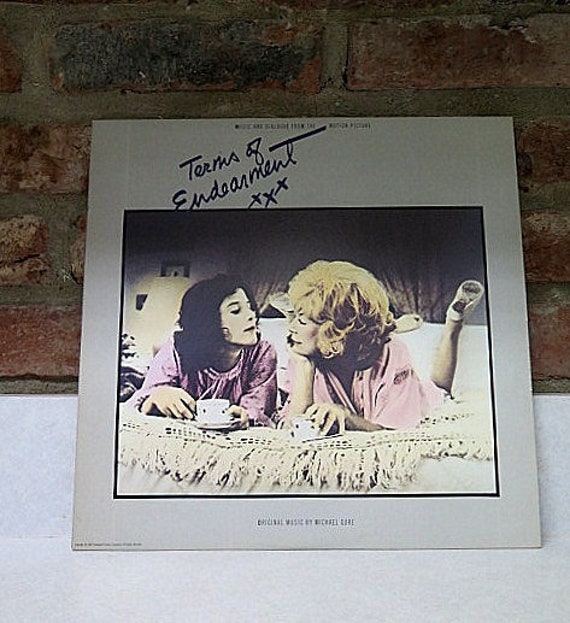The color photo features a vinyl record standing upright and leaning against a brick wall. The bottom of the image reveals a light gray floor. The record sleeve predominantly displays purples and grays, with a photograph at the center depicting Debra Winger and Shirley MacLaine. The two actresses are laying on a tasseled bedspread, facing each other with their feet playfully in the air, capturing an intimate and cheerful moment. This central image is reminiscent of a retro scene, with the women seemingly sharing tea and smiles. At the top of the record sleeve, the text reads "Terms of Endearment XXX," referring to the movie they starred in. Smaller, illegible text is also present both at the top and bottom of the sleeve. The overall composition places the record centered in the photo, with the gray floor and the brick wall making up the background.